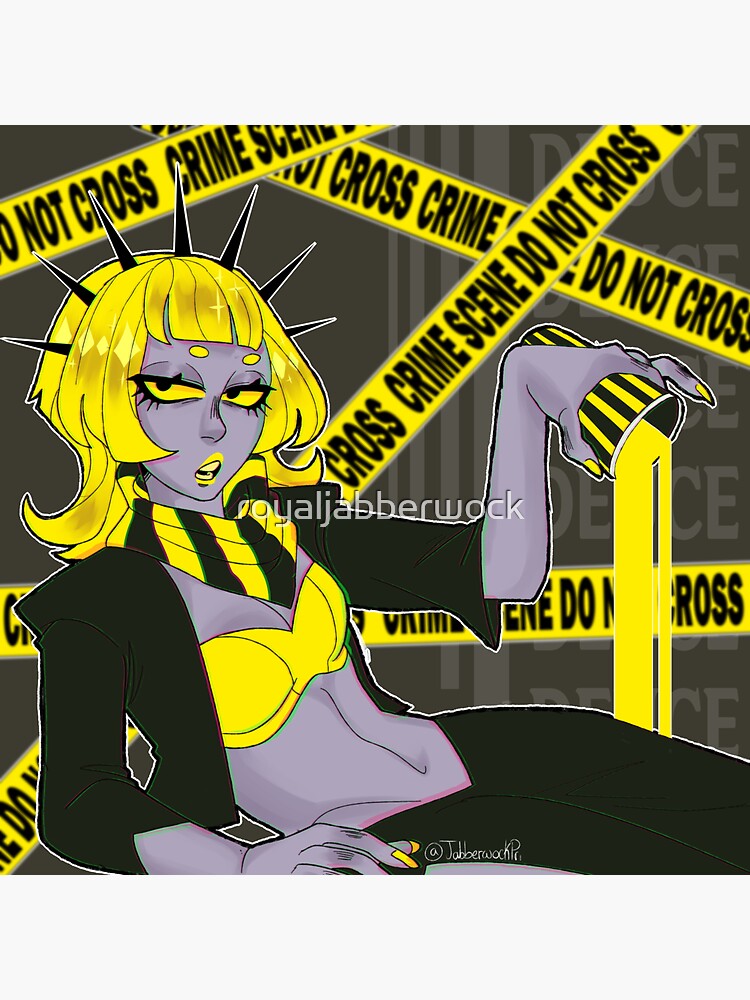The image is a cartoon-style depiction of a woman with a distinctive gray-purple skin tone and an overall striking yellow color scheme. She is leaning on her right elbow, gazing and talking towards the right. The woman is notable for her yellow hair, yellow eyes, and yellow lips. She is dressed in a black jacket or cardigan, a yellow bra, and black pants. Adding to her unique appearance, she wears a black and yellow striped scarf and has sharp black spikes on her head that are reminiscent of the Statue of Liberty's crown.

In her right hand, she holds a black and yellow striped cup from which she pours a yellow liquid. Her fingernails are also painted yellow. The background features bright yellow "Crime Scene, Do Not Cross" tape, reinforcing the theme of a crime scene setting. Despite the vibrant colors and dramatic elements, her facial expression appears bored and disengaged, adding a layer of intrigue to the image.